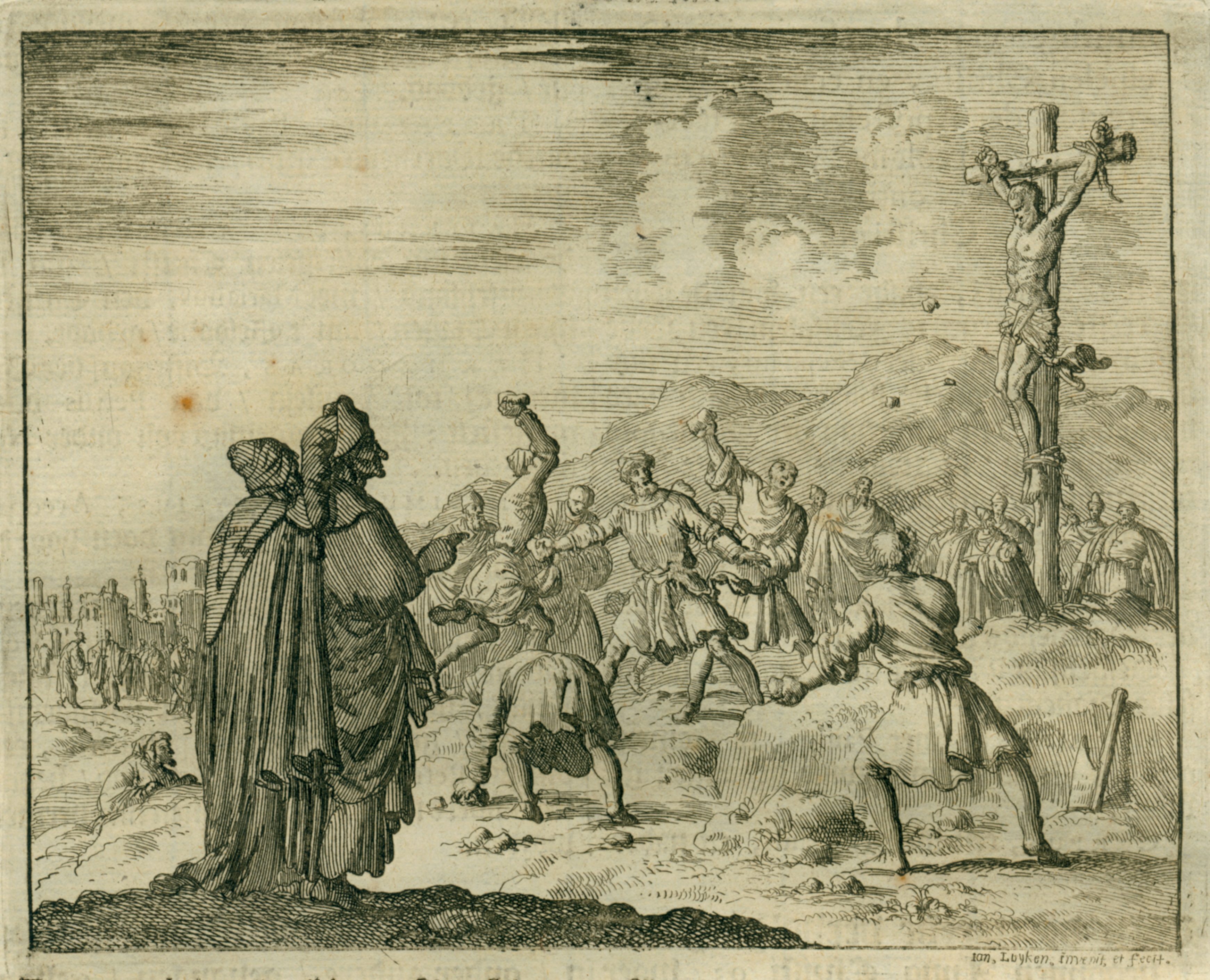This detailed black-and-white sketch appears to be taken from a book and presents a harrowing scene outdoors, likely in the middle of the day given the visibility and detailing of the surroundings. In the top right corner of the image, a man, resembling Jesus, is tied to a cross with a cloth wrapped around his loins, his arms extended above his head and his legs tied at the ankles. Positioned centrally in the image, a group of approximately 20 individuals is depicted hurling rocks towards him, emphasizing the tumultuous aggression of the scene. 

In the foreground, two covered women stand, seemingly observing the distressing action. The background reveals mountains and a cloudy sky, adding a sense of desolation and grandeur to the overall scene. Notably, an off-white border encapsulates the entire image, and a small text or possibly the artist's signature is located at the very bottom. The intricate detailing in shades of black, white, and gray enhances the stark and somber tone of the illustration, which is crafted in a meticulous hand-drawn style.